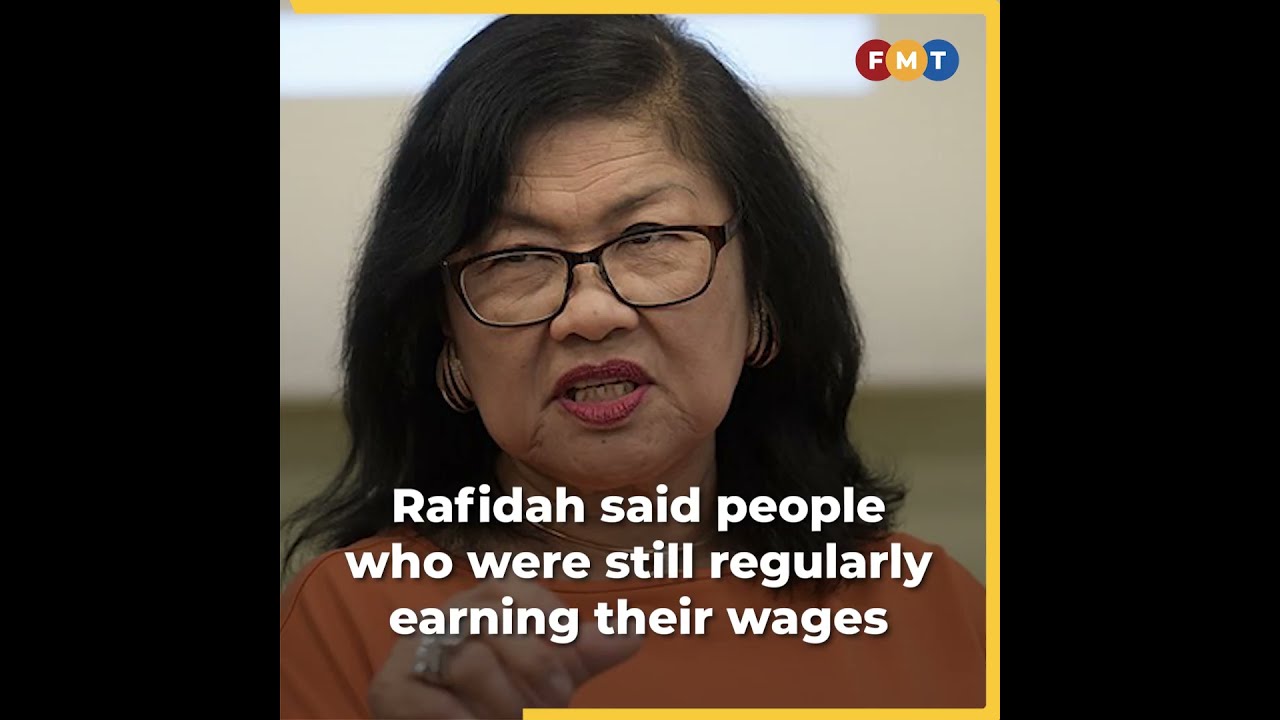In this image, we see a middle-aged woman of Asian descent, likely in her 50s or 60s, with shoulder-length dark brown hair, styled neatly. She is wearing black-framed glasses and has gold earrings in both ears. The woman is donned in an orange, pumpkin-colored top and appears to be speaking, possibly in the midst of a presentation or conversation. Her mouth is slightly open, and her facial expression suggests she might be admonishing someone or emphasizing a point. She is standing against a beige background with a blurred window or light source at the top, contributing to the room's setting.

On the image, there is some text that reads: "Rafida said people who were still regularly earning their wages," indicating that it might be a caption or a transcript of what she is saying. The picture is bordered by a yellow frame, further outlined with black rectangles on the left and right sides. In the upper right-hand corner, the initials "FMT" are prominently displayed within three colored circles: a red circle containing "F," a yellow circle with "M," and a blue circle featuring "T." This emblem may hint at the source or context of the image. Additionally, on her ring finger, the woman is wearing a notably large ring.